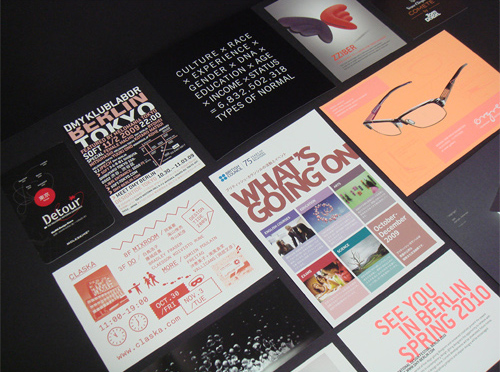The image showcases an organized arrangement of various posters and magazine pages displayed on a black background, resembling a masonry-style grid. At an angle, these elements form a visually cohesive and eclectic collage, mixed with vibrant colors and monochrome designs. In the center, a prominent poster asks, "What's Going On?" Surrounding it, other notable features include a black sign with the text, "Culture, Race, Experience, Gender, DNA, Education, Age, Income, Status, 6,832,502,318 types of normal." Adjacent posters mention "Berlin Tokyo" and display dates like "Spring 2010." Among these, there's an eye-catching orange-y sherbet-colored ad featuring glasses, with a tagline reading, "See You in Berlin, Spring 2010." Another flyer advertises "classica.com," possibly featuring an image resembling a building. The design elements and diverse styles of the pages suggest they're from magazines, arranged meticulously to highlight a variety of themes and visual aesthetics.